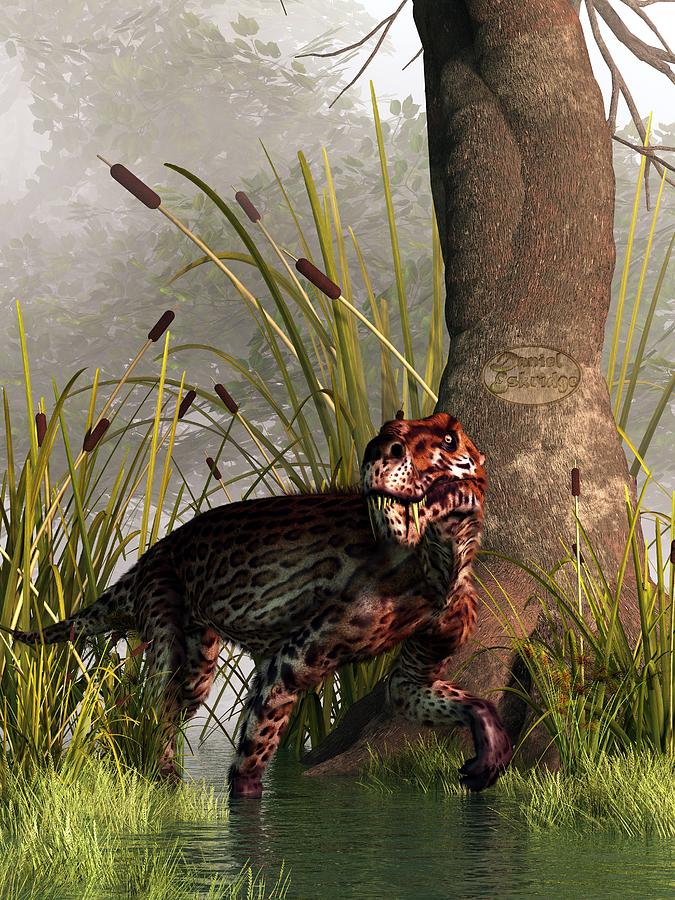The image appears to be a detailed piece of digital art or a hyper-realistic painting depicting a hybrid dinosaur with cheetah-like spots, potentially a T-Rex or similar theropod, navigating through a murky, swampy area. The dinosaur's body is primarily dark, adorned with distinctive leopard-like spots in shades of brown and beige, creating a striking contrast. Its mouth is closed, but sharp teeth protrude from the lower jaw, and one eye is visible, seemingly focused on an unseen object.

The surrounding environment includes a large, imposing tree trunk with a barely discernible logo or artist's signature etched into it. The swamp water is a deep, dark green, accentuated by emergent green plants that punctuate the scene. The background is dense with additional foliage and shrouded in a heavy mist, enhancing the mysterious and eerie atmosphere. No text or people are present in the image, suggesting it might be a screenshot from a 3D animated video or a game.